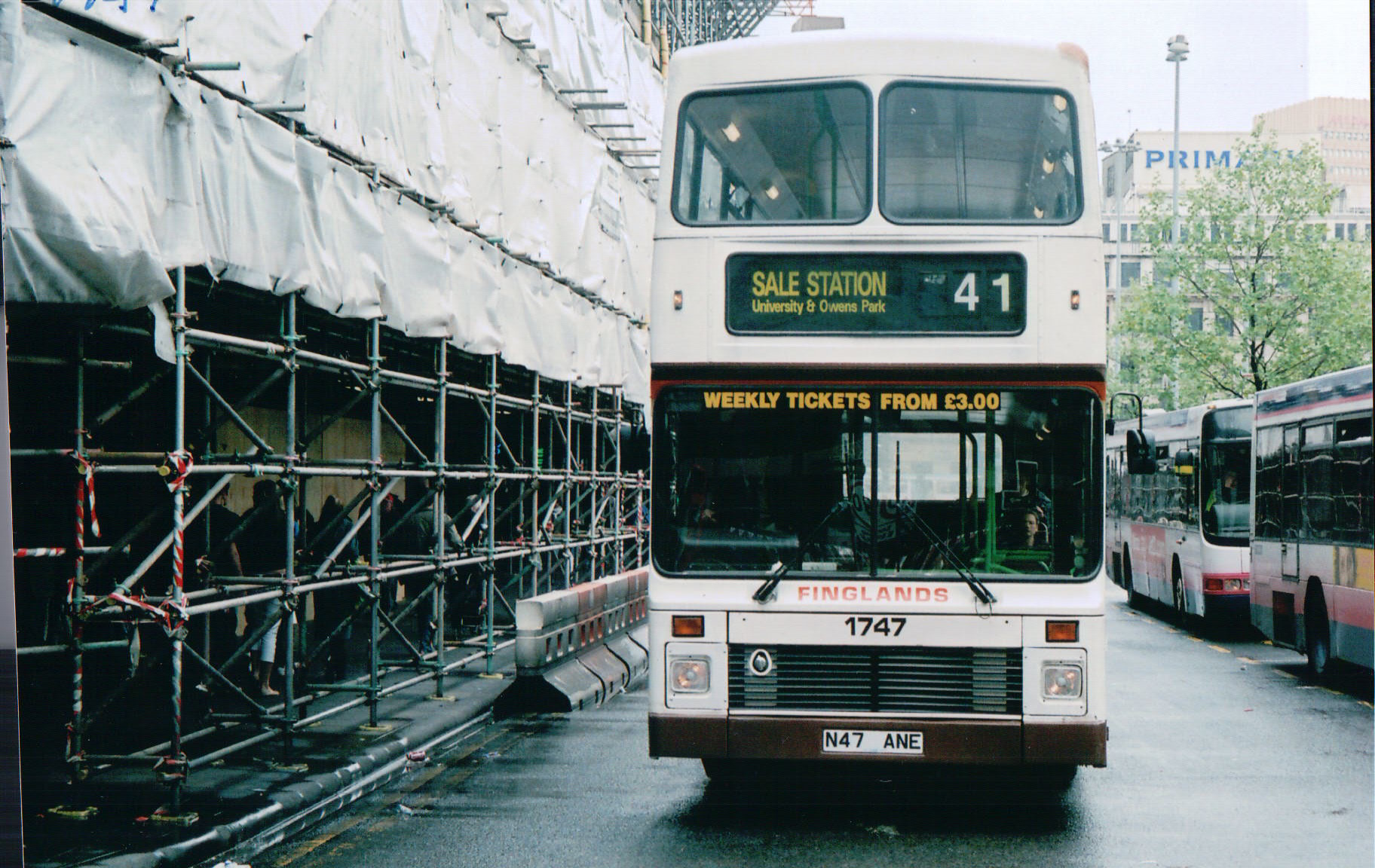In this detailed city scene, a white double-decker bus numbered 41 is approaching the camera. The front sign on the bus displays "Sale Station, University, and Owens Park," and above the large windshield, there's an advertisement for "Weekly tickets from £3." Below the windshield, the name "Finglands" is prominently displayed, followed by the bus number "1747" and the license plate "N47ANE." The driver is visible on the right-hand side of the bus, though no other passengers can be seen. To the right of the street, several other buses are lined up, but they are not double-deckers. The left-hand side reveals a construction area with scaffolding and white tarp covering the sidewalk. In the far background, partial views of buildings can be seen under a grey sky that suggests recent rain. The scene is bustling with people, possibly at the end of the workday, walking beneath constructed awnings beside the scaffolding. Notably, a large building with the letters "P-R-I-M" is visible in the distance, hinting at a store's name.